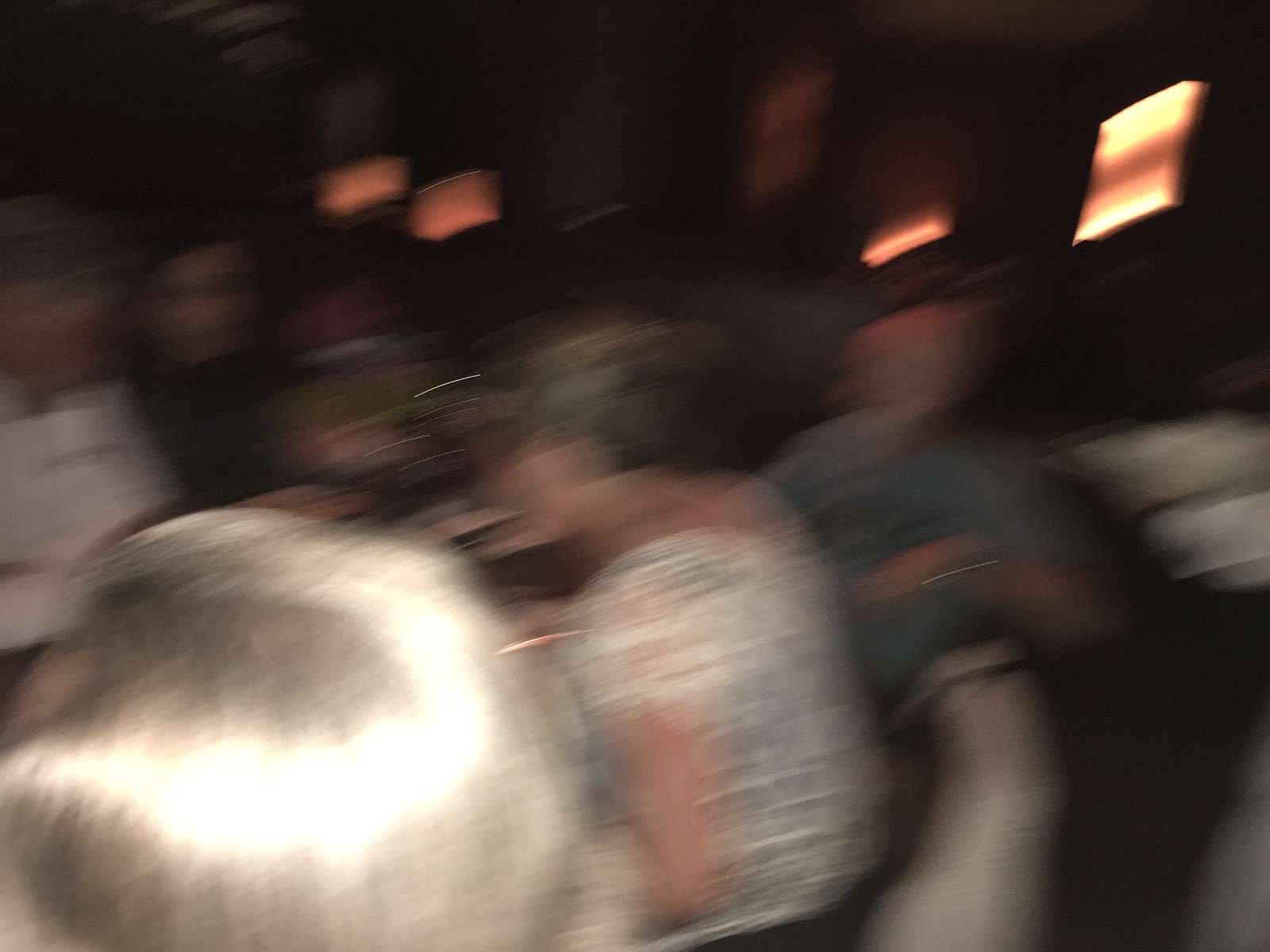A square-shaped, low-resolution image featuring a blurry and pixelated view of several people in a dimly lit setting. Central to the image is an individual facing left, clad in a white top with visible arms. To their immediate right, another person can be discerned amidst the indistinct figures. The bottom left corner reveals the head of yet another individual, with additional people present on the far left side of the frame. The background is predominantly dark, creating a stark contrast with an orange light shining from the top right corner, casting a soft glow over the scene.